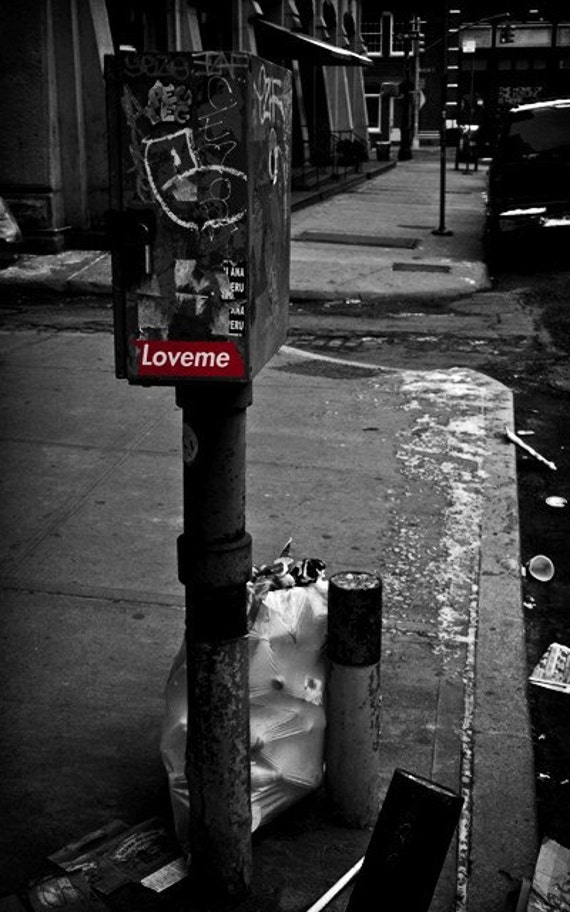In this black and white photograph, the central subject is an old, graffitied payphone or mailbox positioned slightly to the left of center on a gritty, snow-dusted sidewalk. The metal structure is marked with various white graffiti and signs of rust. The only splash of color in the entire image is a vivid red sticker with the words "LOVE ME" in white text. Surrounding the payphone are piles of trash, including paper cups, straws, and two white trash bags resting against small pylons or poles. The background reveals tall buildings characteristic of a cityscape, with a car visible on the street and stone-like tiles adorning the exteriors of the buildings. The street itself has a brick or cobblestone appearance, reminiscent of a New York City street in Brooklyn. The scene evokes a stark, cold, and somewhat deserted urban environment, captured in winter with a dark and high-contrast photographic style.